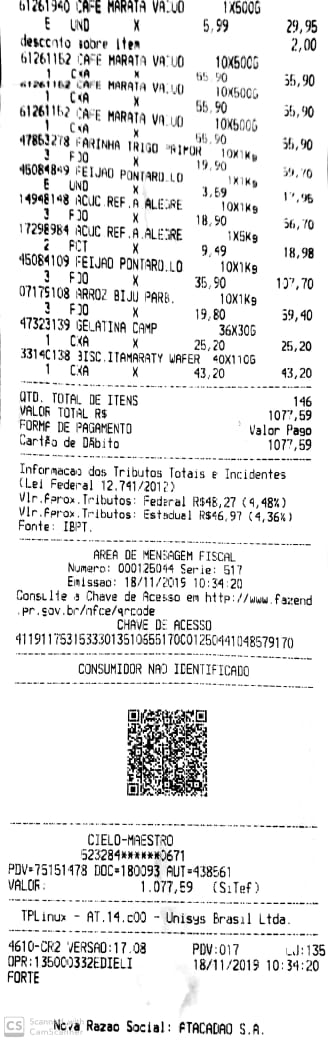The image shows a close-up scan of a long, rectangular grocery store receipt written entirely in Italian, featuring black ink on white paper. The top half of the receipt lists numerous purchased items, including names and prices, such as "Wafer" and "Allegre," with possibly some Italian Martini and wine products. Below the detailed items, separated by dashed lines, is the total amount of the items, followed by what appears to be tax information with percentage signs like 4.48% and 104.36%. Toward the bottom of the receipt, below the totals, there is a section that possibly contains date and time details. Near the very bottom, there’s a QR code. The footer of the receipt includes partially readable text “Nosa social” and a business name, "Atacado SA," which may indicate a South American origin. The entire receipt is presented in monochrome.